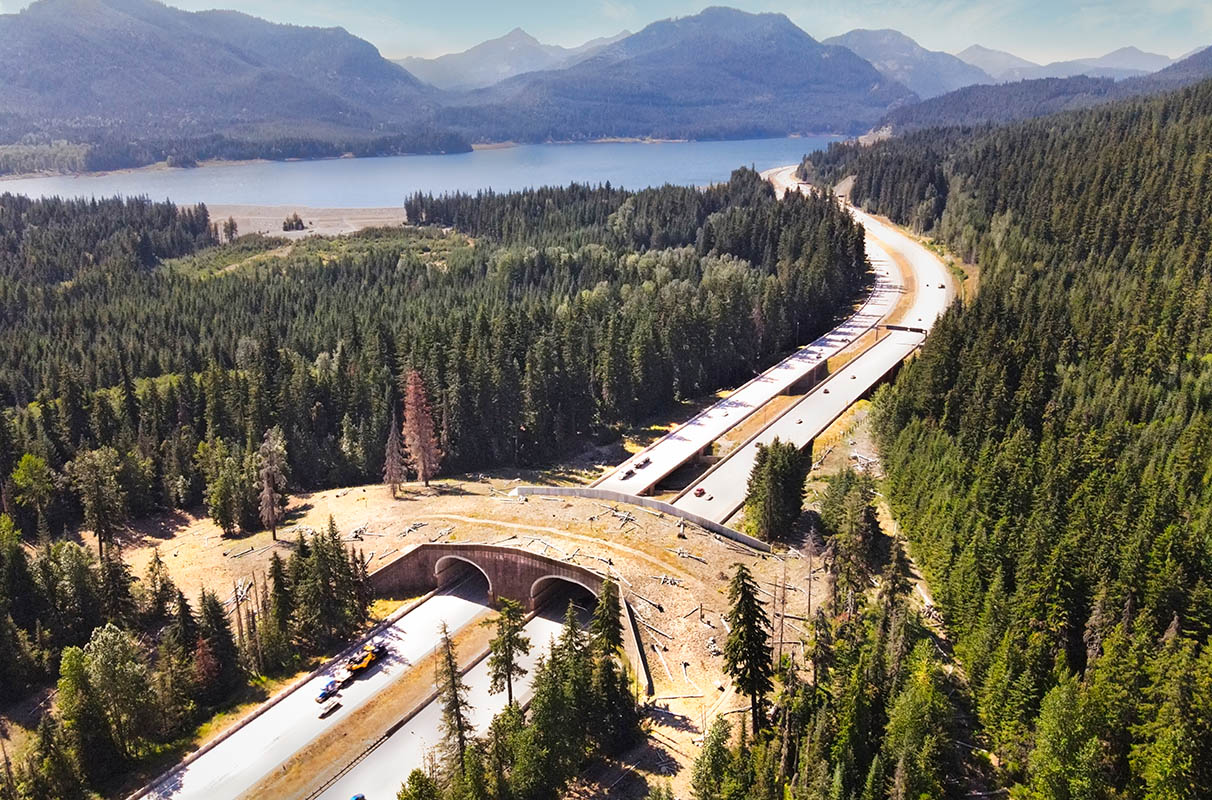The aerial image captures a silver-colored, two-lane highway cutting through a vibrant landscape. The highway originates at the bottom left of the image and stretches towards the top right. Midway through its path, it passes beneath a large, brown bridge, which appears to be under construction with visible patches of dirt and makeshift pathways crossing over it, hinting that wildlife might still use this space. The bridge features two tunnels in alignment with the lanes of the highway.

Flanking the highway on both sides are dense forests of green pine trees. On the right side of the image, these evergreens appear particularly vibrant, while they seem slightly darker on the left. In the distance, beyond the lush forests, lies a serene blue lake, which extends up to a range of dark brown mountains in the upper part of the image. Looming above these mountains, a dark blue sky completes the scene.

Interspersed along the highway are various cars of different types and colors, moving along their routes. The overall texture of the landscape, from the vibrant greens of the forest to the earthy tones of the bridge and the cool blues of the distance, yields a richly detailed and dynamic view.